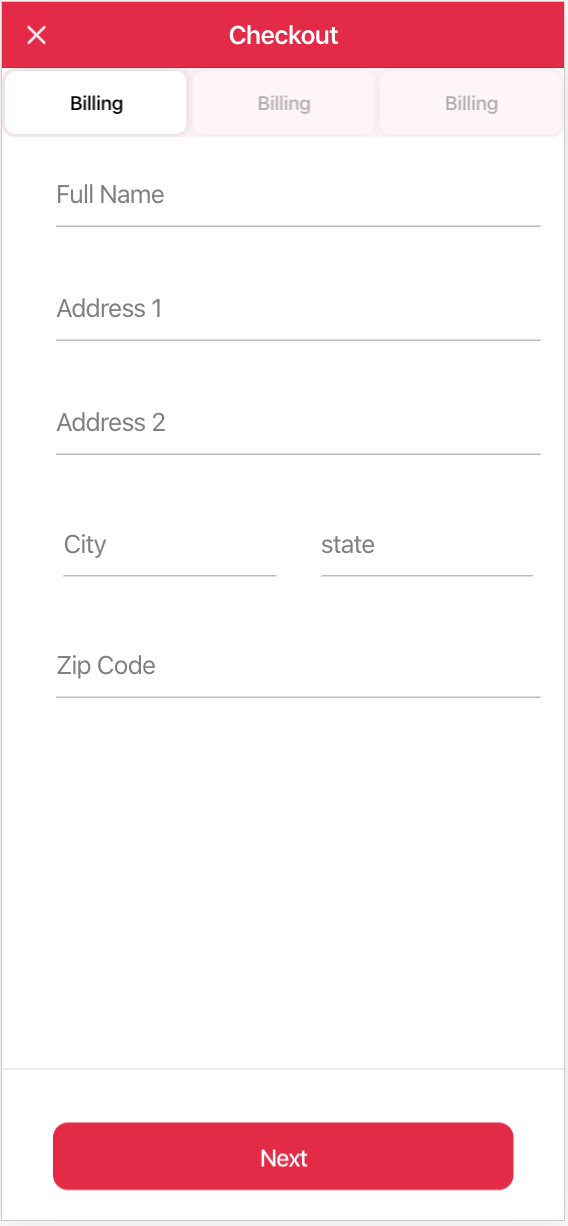The image portrays a largely blank checkout page. Centered at the top, a prominent red rectangle displays the word "CHECKOUT" in bold white letters, accompanied by a white "X" on the left side, likely indicating an option to close the page. Below this, three squares labeled "BILLING" are aligned horizontally, with the leftmost square highlighted in a brighter shade of white, signifying the active section.

Directly beneath, a series of text fields are presented for user input. The first field, labeled "FULL NAME," is followed by "ADDRESS 1" and "ADDRESS 2." Subsequent fields prompt the user to enter their city and state, and finally, their zip code. At the bottom of the page, a clickable red rectangle features the word "NEXT" in white letters, designed to advance the user to the following page once all required information is provided.